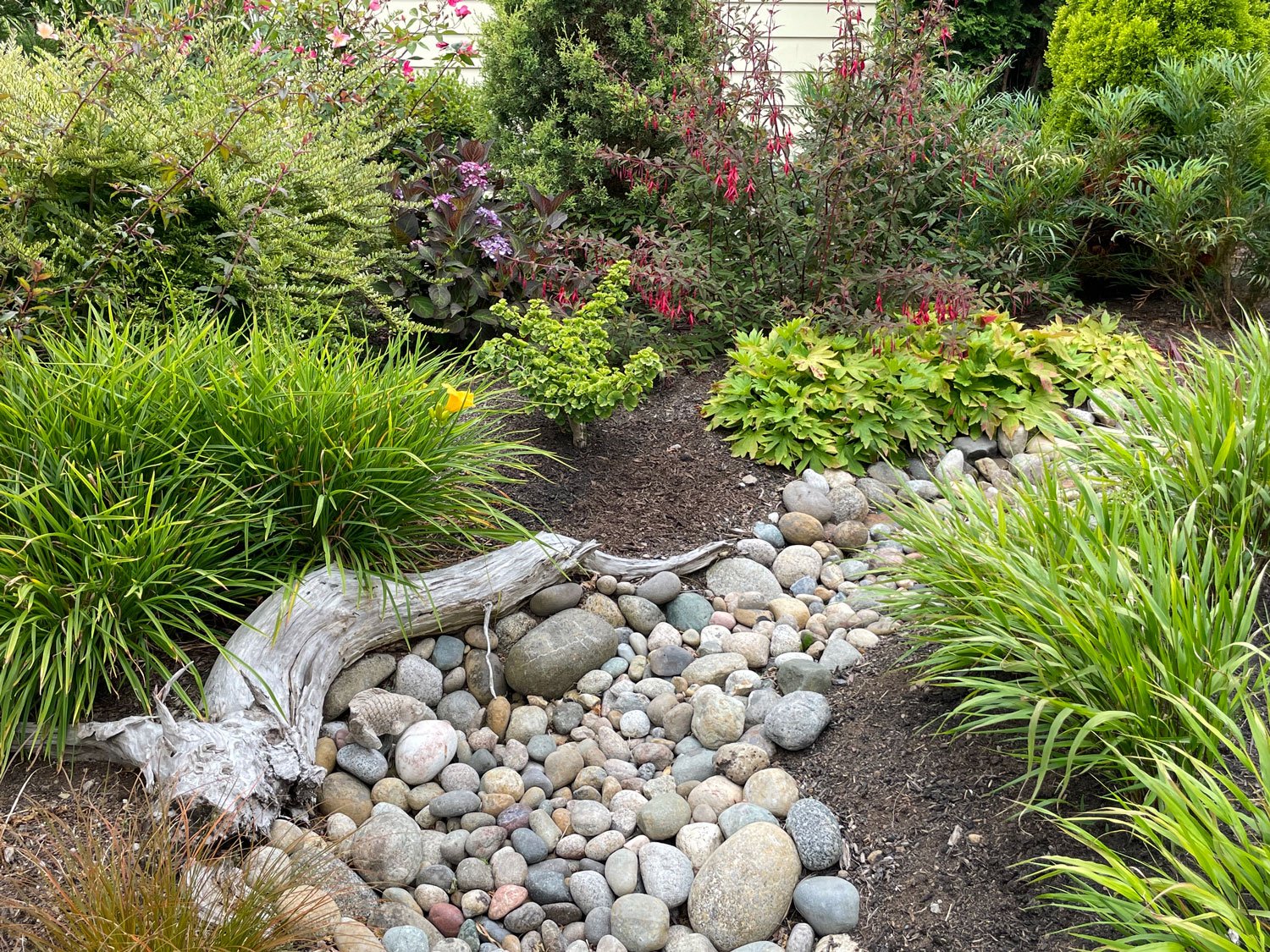This daytime outdoor photograph captures a backyard or side yard area, likely of a residence, with a mix of well-maintained and overgrown garden features. In the foreground, there's an expansive bed of river rocks in varied colors—white, pink, light blue, and beige—forming a path that narrows as it extends. Among these rocks, a piece of driftwood lies along the left side. The garden areas feature a combination of dark brown soil and woodchipped sections with various green shrubs and a few scattered weeds. Splashes of vibrant red, purple, and pink flowers add contrast to the predominantly green foliage. Towards the back, dense trees create a leafy backdrop near the house, which is partially visible and severely cropped. The right side of the image shows clustered green plants, creating a lush, though slightly wild, atmosphere. In the bottom left corner, some brushed grass peeks into the frame, accentuating the natural, somewhat untamed setting.